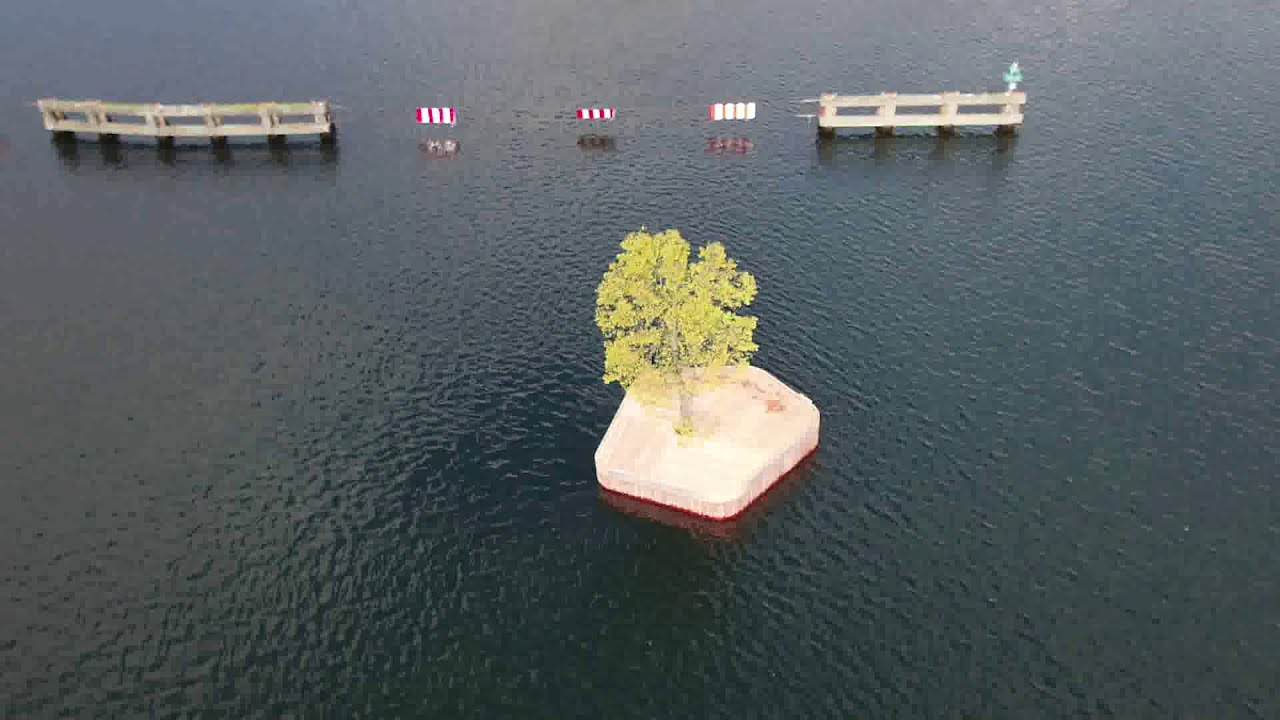The image is a horizontally aligned rectangular picture taken from a very high angle, looking down at a body of dark bluish-gray water with gentle ripples. In the center of the image, there's a small, white cement island shaped like a pentagon with rounded edges, approximately 30 feet across. The island features a single, medium-sized tree with bright green leaves. Surrounding the island are some red markings at its base.

In the background, the water stretches across the majority of the photo. There are two concrete structures protruding from the water, reminiscent of remnants from a previous building. Between these structures, there are three vertically striped red and white banners tied on strings. Additionally, wooden fence-like barriers with multiple rectangles are visible in the upper left and right corners of the image, further emphasizing the textured, calm water and creating a visual frame around the central island.